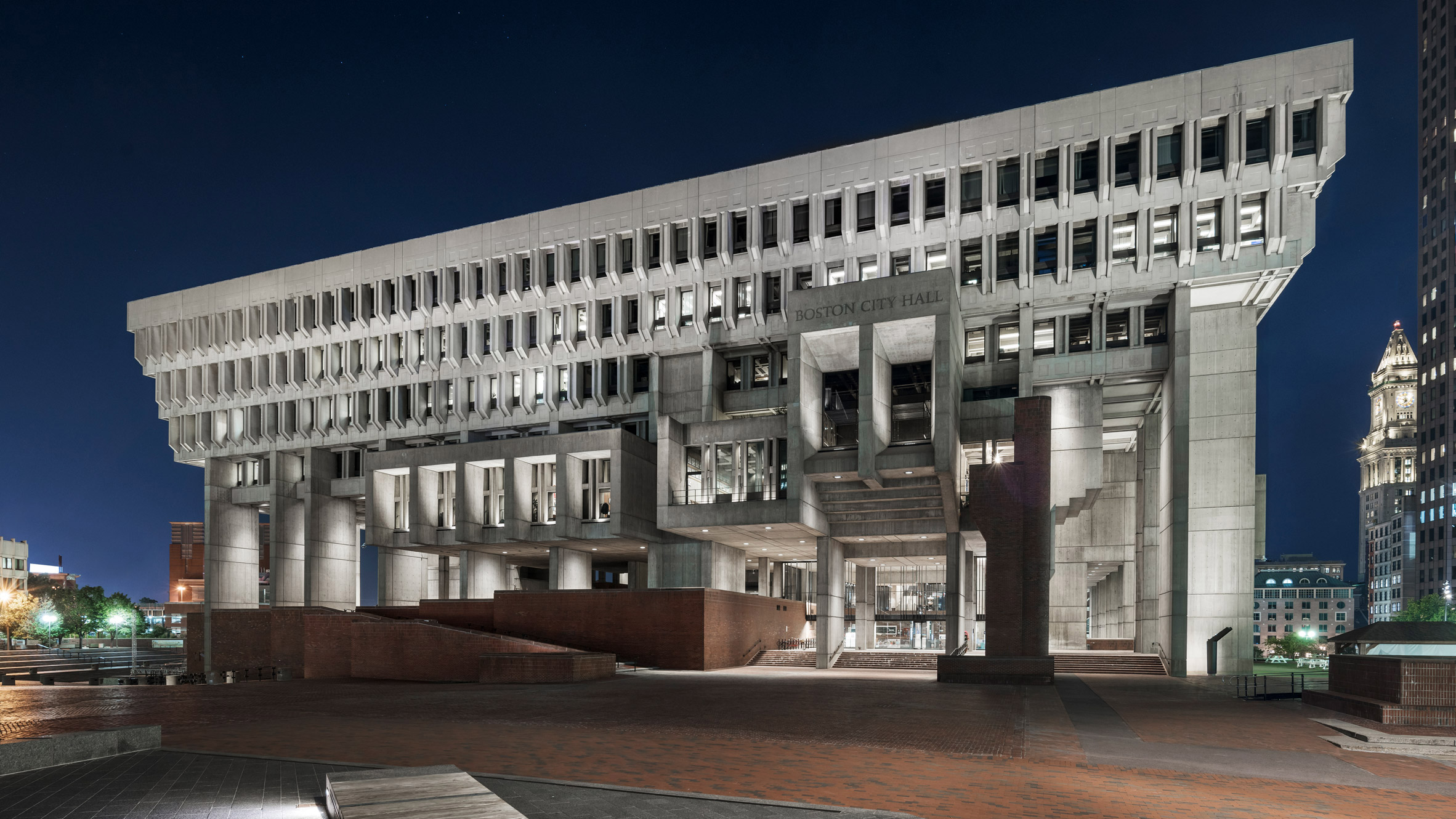The image showcases an outdoor nighttime view of the Boston City Hall building from a side perspective at street level, approximately 20 feet away. The building, constructed of gray cement, exhibits a modern, inverted step pyramid design, where each upper story juts out further than the one below. The structure is five stories tall with a glass door entrance on the first floor. Above the entrance, the words "Boston City Hall" are etched into a protruding concrete section with two window cutouts. The facade features numerous rectangular windows, some lit, some dark, distributed across three distinct levels. The red and brown brick walkway in front of the building adds contrast to the stone facade. Flanking the City Hall, on the left and right, are lit-up buildings of varying heights, hinting at the surrounding cityscape. The dark blue night sky frames the scene, adding to the atmosphere. In the background, a few distant trees and additional buildings, including a tall skyscraper, are partially visible.